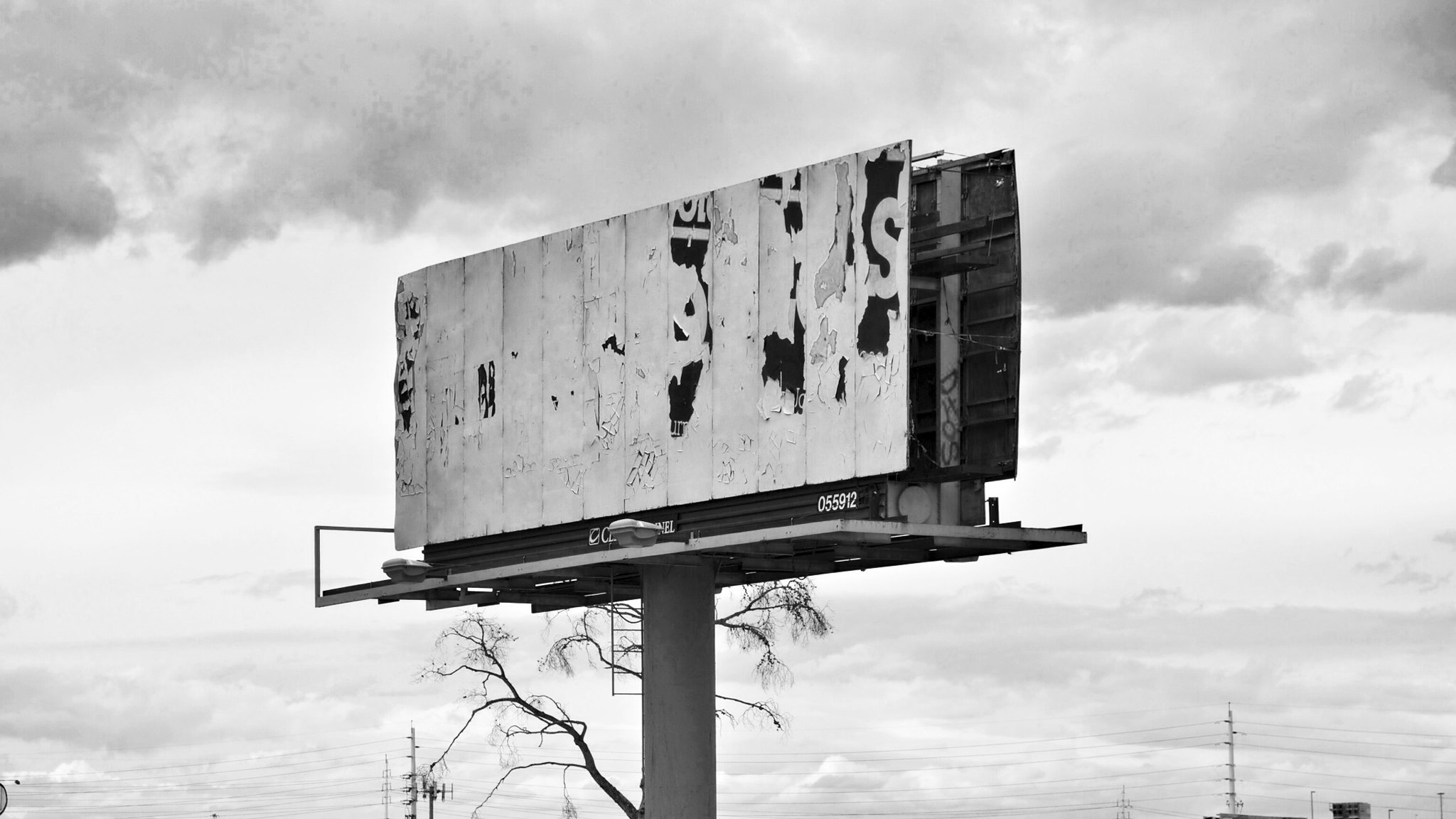In this black-and-white photograph, a cloudy and gray sky looms overhead, creating an overall sense of dreariness and desolation. Toward the horizon, a series of power lines stretch horizontally, and at the bottom of the frame, you can see a few transformer poles bristling with wires. Dominating the foreground is a large, thick metal pole that supports a rectangular, weather-beaten billboard. The billboard, which features a ladder and a catwalk on the front and back, is equipped with lights for illumination. However, the advertisement that once graced the billboard is now torn and unrecognizable, with only a few strips of paper clinging stubbornly, including a noticeable 'S' in the upper right-hand corner. Behind the billboard, a leafless, skinny tree adds to the scene's somber atmosphere, reinforcing the overall feeling of abandonment and decay.